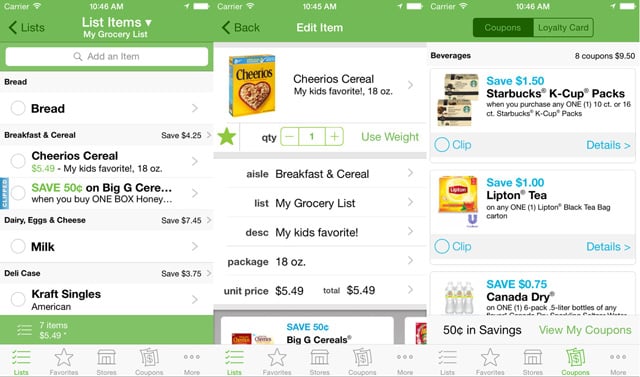The image depicts a mobile shopping application displayed on three adjacent phone screens. The top part of each screen shows the status bar, indicating the carrier, Wi-Fi signal strength, the time (10:40 AM), full battery icon, and other standard notifications. The header section is green with white text, displaying "Lists" and a back button in black. 

The primary screen showcases a grocery list titled "My Grocery List," beneath which is a search bar with placeholder text "Add an item." Listed items include "Bread," with radio buttons for selection, and a more detailed entry: "Cheerios Cereal" marked as "$5.49 - My kids' favorite, 18 ounces, with 50 cents off on purchasing one box of honey cereal."

Additional categories like "Dairy, Eggs, and Cheese" feature savings details, such as "Save $7.45 on milk" and "Save $3.75 on Kraft Singles American (7 items, $5.49)." At the bottom of the screen, there are tabs labeled "List," "Favorite Stores," "Coupons," and "More."

The subsequent screens appear to delve deeper into the items, reiterating details like "Cheerios Cereal - My kids' favorite, 18 ounces" with a quantity of "1." These screens provide options to categorize the item under "Breakfast Food" and tags such as "my list" and "my groceries," emphasizing the personalized nature of the shopping experience.